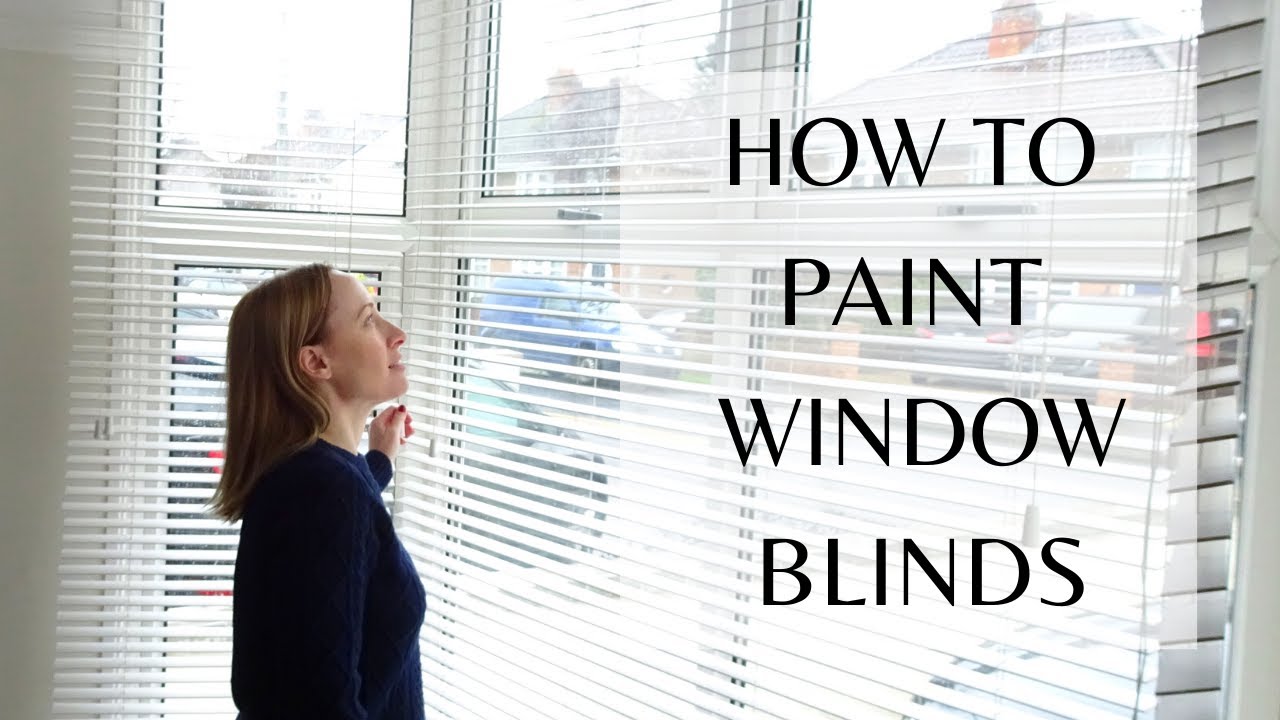In this image, a clear and concise instructional guide reads "How to Paint Window Blinds" in bold black letters on the right side, making it easily readable. The centerpiece of the image is a white woman with shoulder-length reddish-brown hair, which is neatly pushed back behind her ear, thus revealing her face. She is standing in her home, facing a set of large, four-pane windows adorned with old-style blinds. She is wearing a blue sweater and focusing her gaze upward at the blinds, with one hand gripping the drawstring, demonstrating the process of opening them. The scene outside the window reveals a calm neighborhood with a road and houses lining the street, and a blue van parked on the sidewalk. Sunlight streams through the windows, adding a warm glow to the composition, while the woman's thoughtful anticipation suggests she is about to begin the project featured in this instructional content.